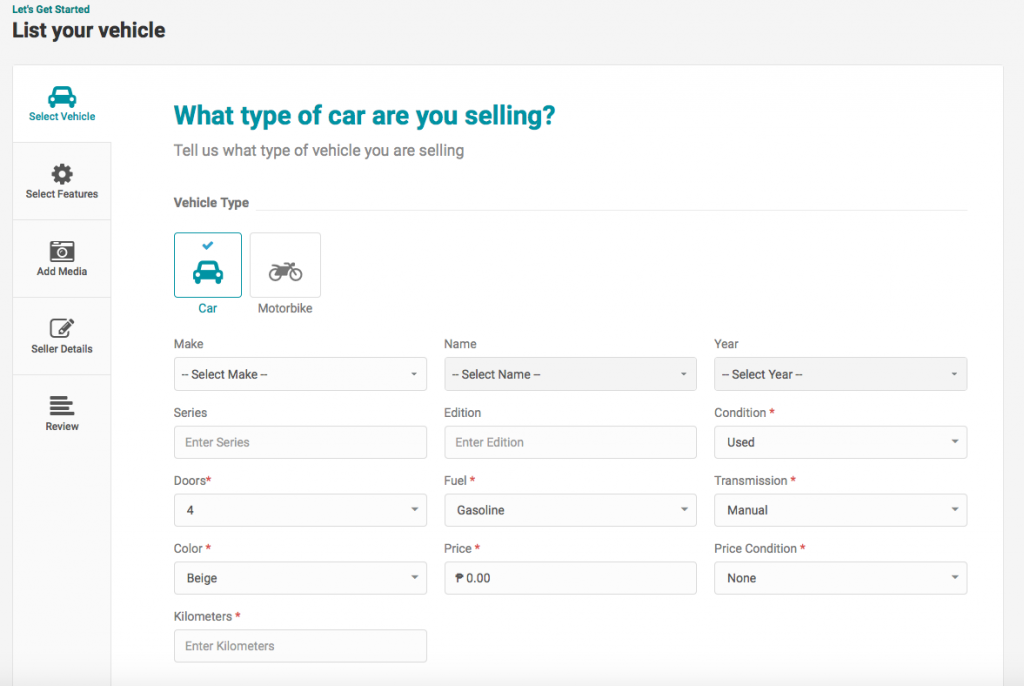The image depicts a webpage with a clean, white background and content displayed in two colors: blue and black. In the top left corner, the phrase "Let's Get Started" is prominently written in blue. Beneath this, in black text, are the words "List your vehicle."

Below this introductory text, there are five selectable boxes arranged vertically. The first box, highlighted with a blue background, features a blue car icon and is labeled "Select the vehicle" in blue text. The second box, outlined in black, features a settings icon and is labeled "Select features" in black text. The third box depicts a camera icon, accompanied by the text "Add media." The fourth box shows a pen icon and is labeled "Seller details," and the final box features a review checkmark icon and is labeled "Review."

To the right of this vertical column, there is text in blue asking, "What type of car are you selling?" Directly beneath this question, written in either black or light gray, is the prompt, "Tell us what type of vehicle you're selling." The following section is labeled "Vehicle type" and offers two options: "Car" and "Motorbike." Below this are approximately twelve drop-down selections for specific vehicle details: make, model, year, series, edition, condition, doors, fuel type, transmission, exterior color, price, and mileage (in kilometers).